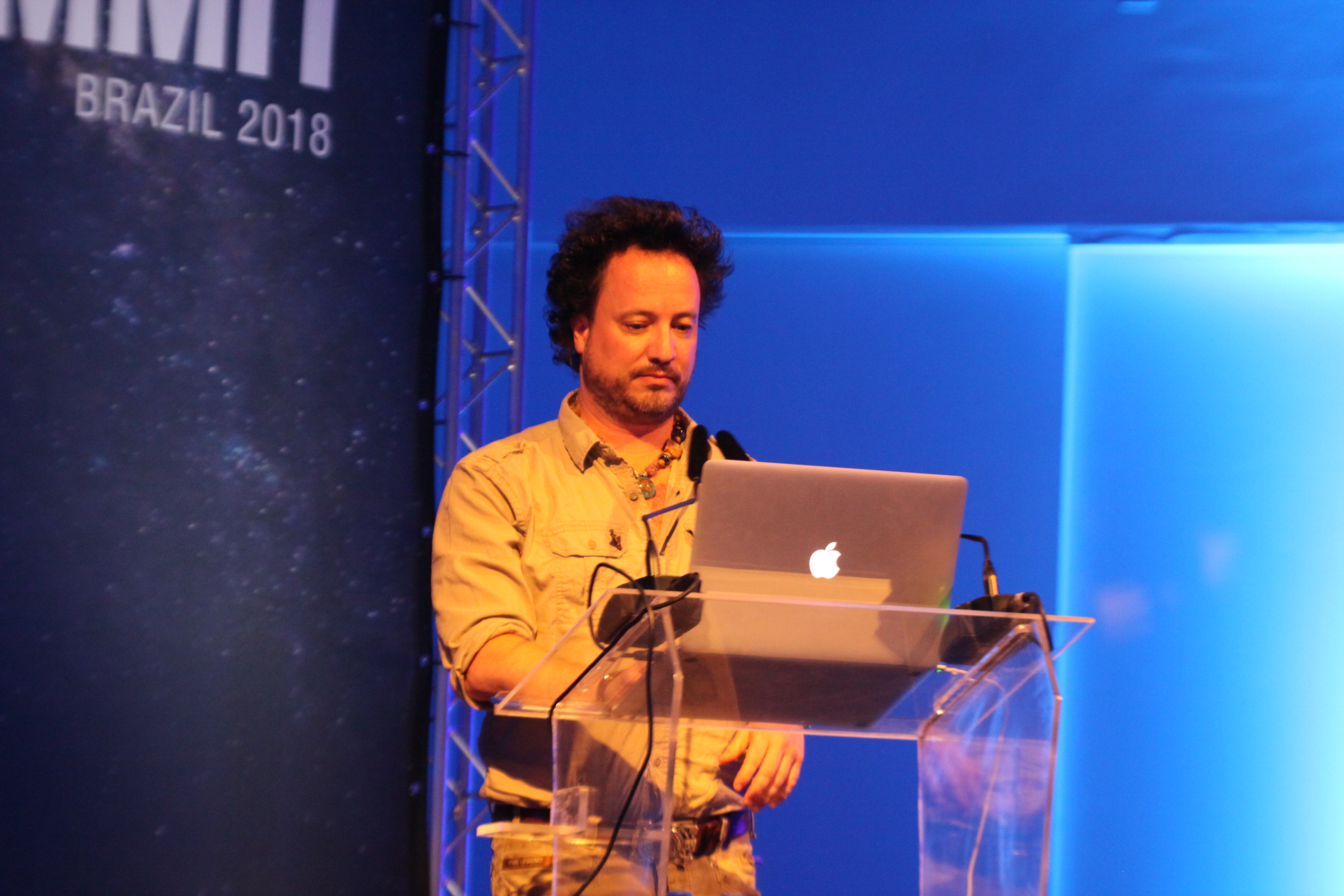The image depicts a Caucasian man standing at a clear acrylic podium during a seminar. The podium has an Apple MacBook with its logo illuminated, flanked by microphones. The man, dressed in khaki pants and a matching button-down shirt with sleeves rolled up to his elbows, sports a dark belt and a chunky beaded necklace. He has short, feathered dark hair, a mustache, and a short beard. His right hand is on the laptop while his left hand rests near his belt. Behind him, the wall features a dark blue cosmic theme with images of galaxies and stars, and the partially visible text "Brazil, space, 2018" is written prominently. The background also includes shades of blue with fluorescent light reflections.